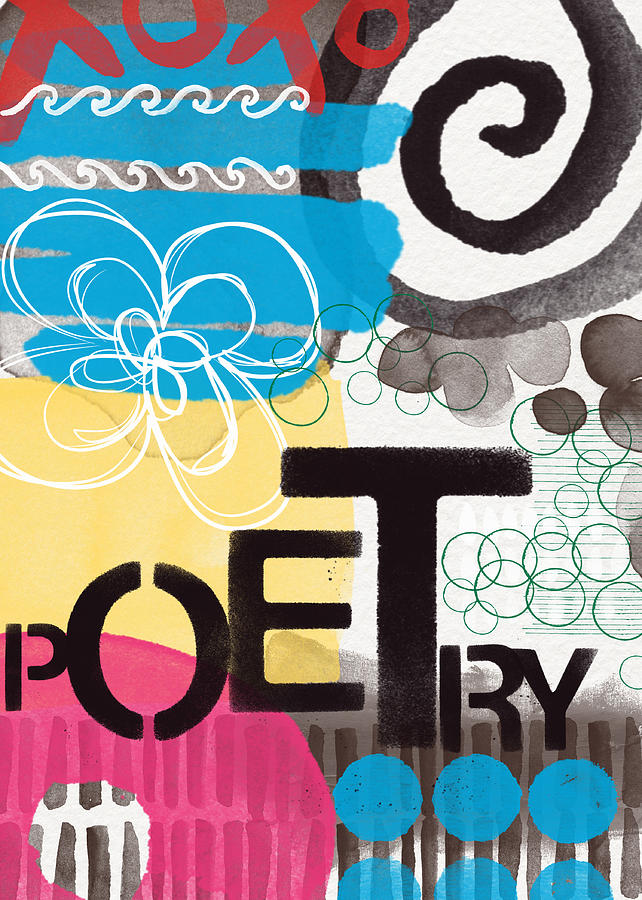The poster is a vibrant piece of abstract art emphasizing the word "POETRY." The orientation is portrait, and it features a variety of colors and patterns. At the very top, the red letters "XOXO" stand out against a blue background in the upper left corner. Just below this, five thick blue lines are visible. Moving to the upper right, there is a black concentric swirl pattern set on a white background. The left side of the poster includes a prominent red circle over a yellow background, and a white wave design can be seen underneath the "XOXO." The right side features an assortment of black and blue circles, beneath the swirl pattern. Notably, the word "POETRY" is creatively arranged in stencil-like, all-caps letters of varying sizes and is positioned starting just below the center on the left. The "P" is smaller and black, followed by a large "O," an even larger "E," a very tall "T," a smaller "R," and "Y," moving through different background hues—from pink to yellow, and finally a white background with green circles. The lower right corner of the poster has blue circles over a black and white striped background, contributing to the overall dynamic and eclectic feel of this artwork.